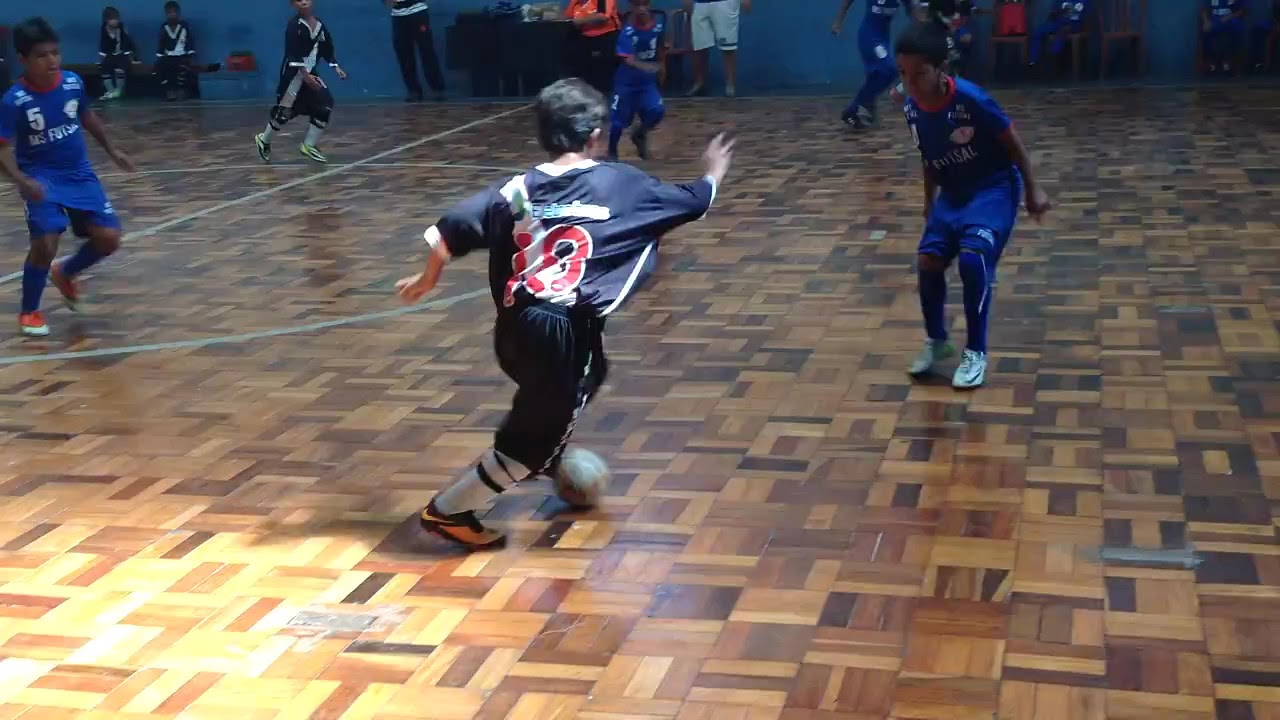In the image, a group of school children is engaged in an indoor soccer game on a gymnasium court with a brown, checkered wood pattern. The children are wearing uniforms primarily in shades of blue; some uniforms feature white and red trim. The focal point is a boy at the forefront, wearing a uniform with the number 19, kicking a small white ball. He has short dark hair and is in mid-motion, with one leg extended back. Around him are other children, clad in similar blue and dark blue uniforms, either running towards him or positioning to interact with the ball. The background reveals a light blue wall and spectators, including adults seated on benches and some standing. A bright light source is visible in the lower left corner of the image, adding a noticeable shine above the scene.